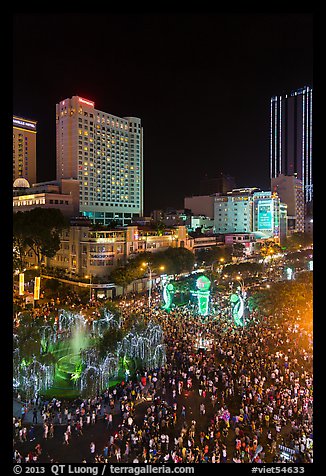The photograph captures a vibrant night-time scene in a city plaza filled with a large crowd eagerly gathered to witness a laser show. The sky is pitch black, indicative of the night setting. In the center of the street, a bright neon green laser hologram draws the crowd’s attention. Surrounding the plaza are towering, well-lit skyscrapers, including one that resembles a hotel, along with other shorter buildings illuminated from within. The image, encased in a black frame, has a white background and includes text at the bottom for copyright information, specifically noting "© 2013 qtluong.com" and a hashtag "viet54633." The entire scene is a blur of lights and movement, emphasizing the dynamic and entertainment-focused atmosphere of a bustling city night.